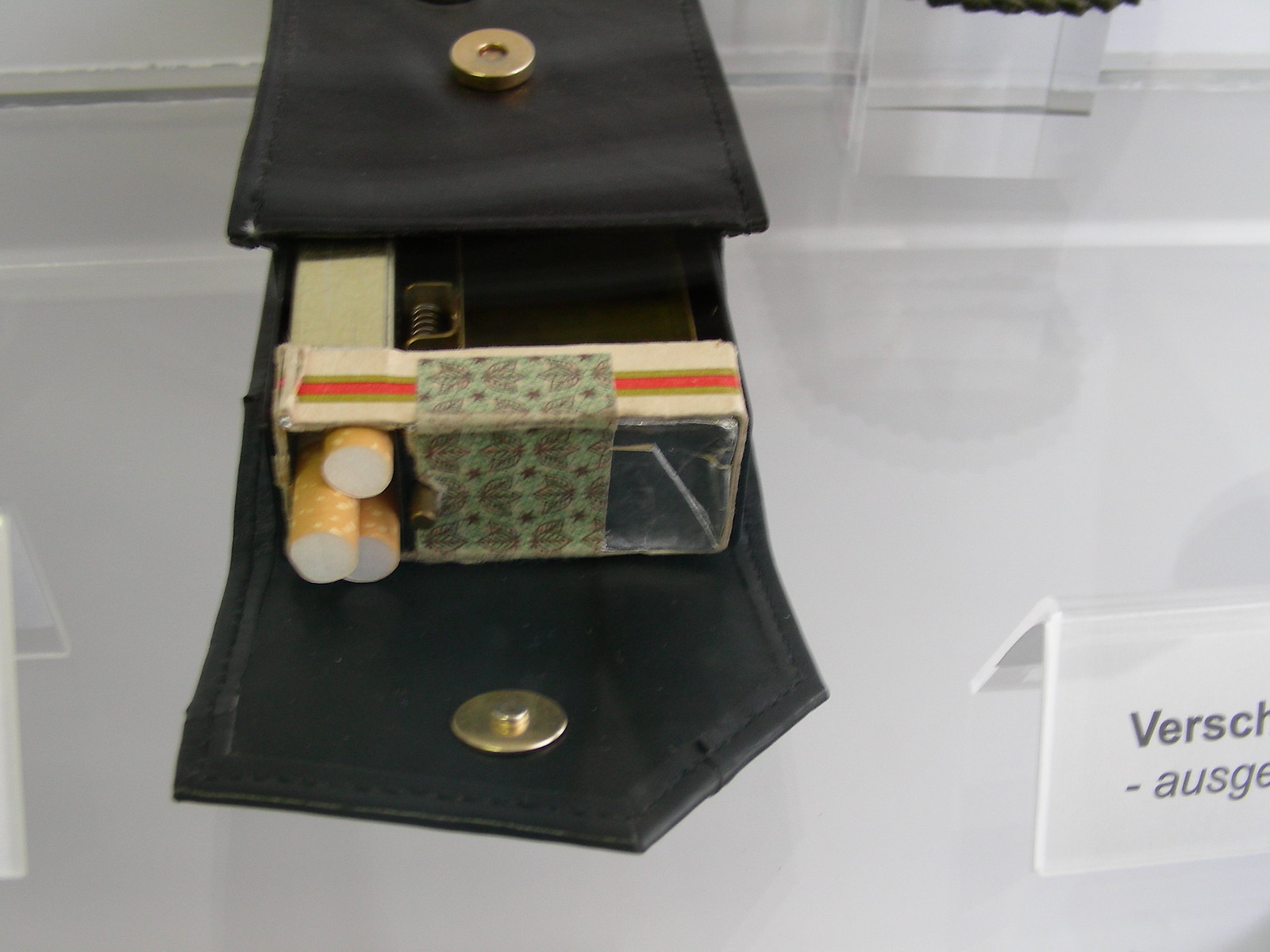The image depicts a black handbag, detailed with visible stitching on the sides, and adorned with gold magnetic snaps at both the top and bottom. The bag is open, revealing the inside at the top of the image. Placed horizontally on its surface is a rectangular, brown cigarette holder with three cigarettes protruding, white with brown tips. The holder features a Gucci-like design, accented by a red line with two holes, and a green sticker in the middle, showcasing a floral motif. Accompanying the handbag, on a white table, is a triangular white card inscribed with text in a language other than English, partially reading "VERSCH" and "AUSGE."